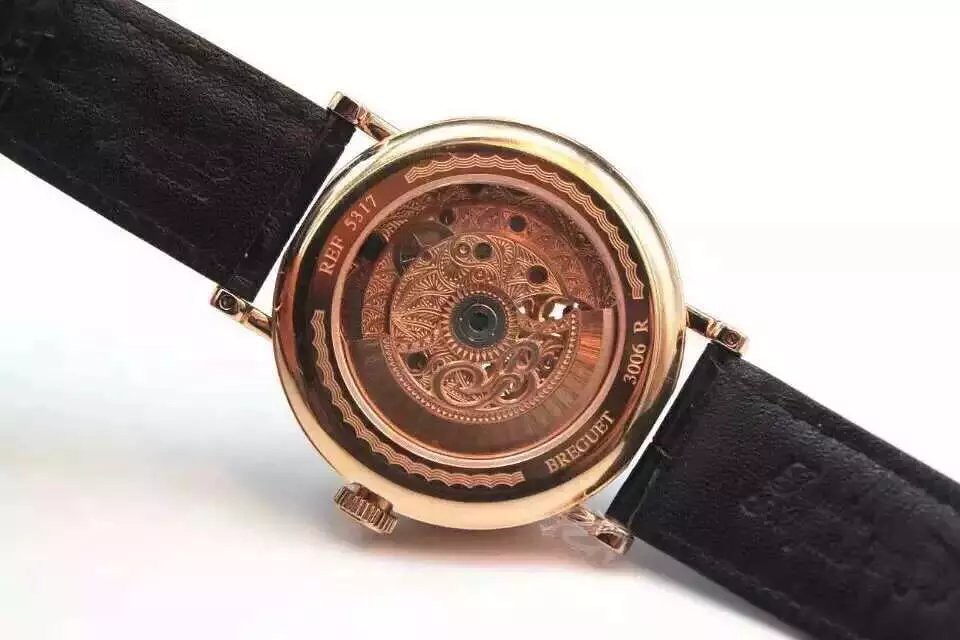The image showcases a zoomed-in, close-up view of a luxury watch set against a white background. The watch itself is positioned diagonally, with the top part angled towards the upper left corner and the bottom part extending to the lower right corner. A portion of the black leather watch band is visible on both sides, although not entirely. The face of the watch is round and primarily a bronze-gold color, displaying a design with intricate, swirly, or wavy lines, particularly in the center, giving it a gear-like appearance. At the top of the watch face, the engraving reads "REF 5317," while the bottom features "3006R" along with the word "BREGUET." The watch does not display any numerical markers for the time, but it does have a visible button likely used for setting the time.